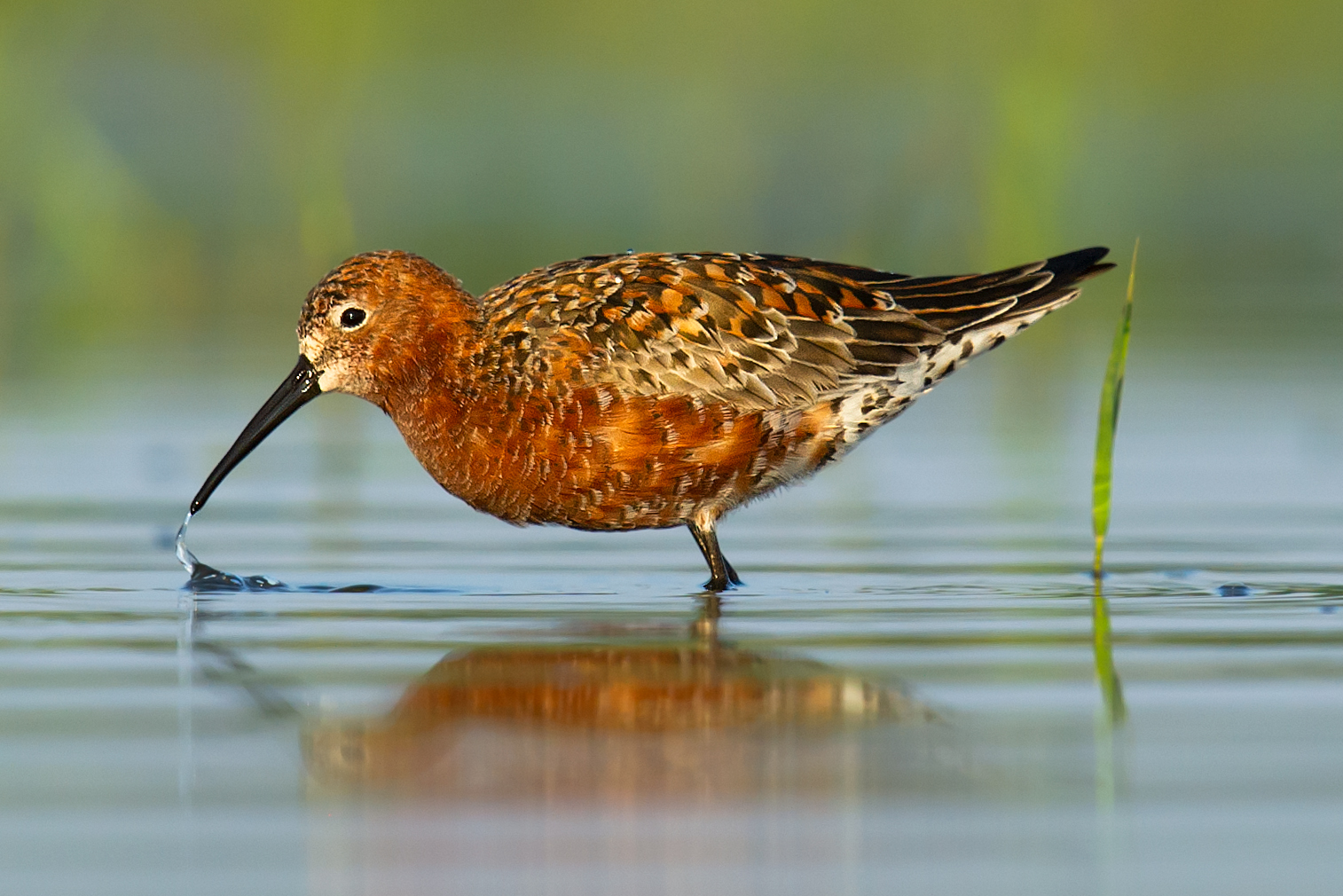This highly detailed photorealistic image, possibly a piece of art or computer-generated imagery, depicts a bird standing in a shallow body of water or a puddle. The bird, which may be either a loon or a snipe, stands facing left, revealing only its left side to the viewer. With legs submerged nearly up to its body, the bird's various shades of brown and black, calico-like plumage contrast with the water's light blue hue. Its long, black beak has just emerged from the water, seemingly holding either a small fish or dripping water. Captured within the water's reflection, the bird stands near a single blade of green grass protruding from the water just behind its tail. The background, blurred with hints of more greenery and plants, subtly emphasizes the shallow water's delicate ripples surrounding the bird.